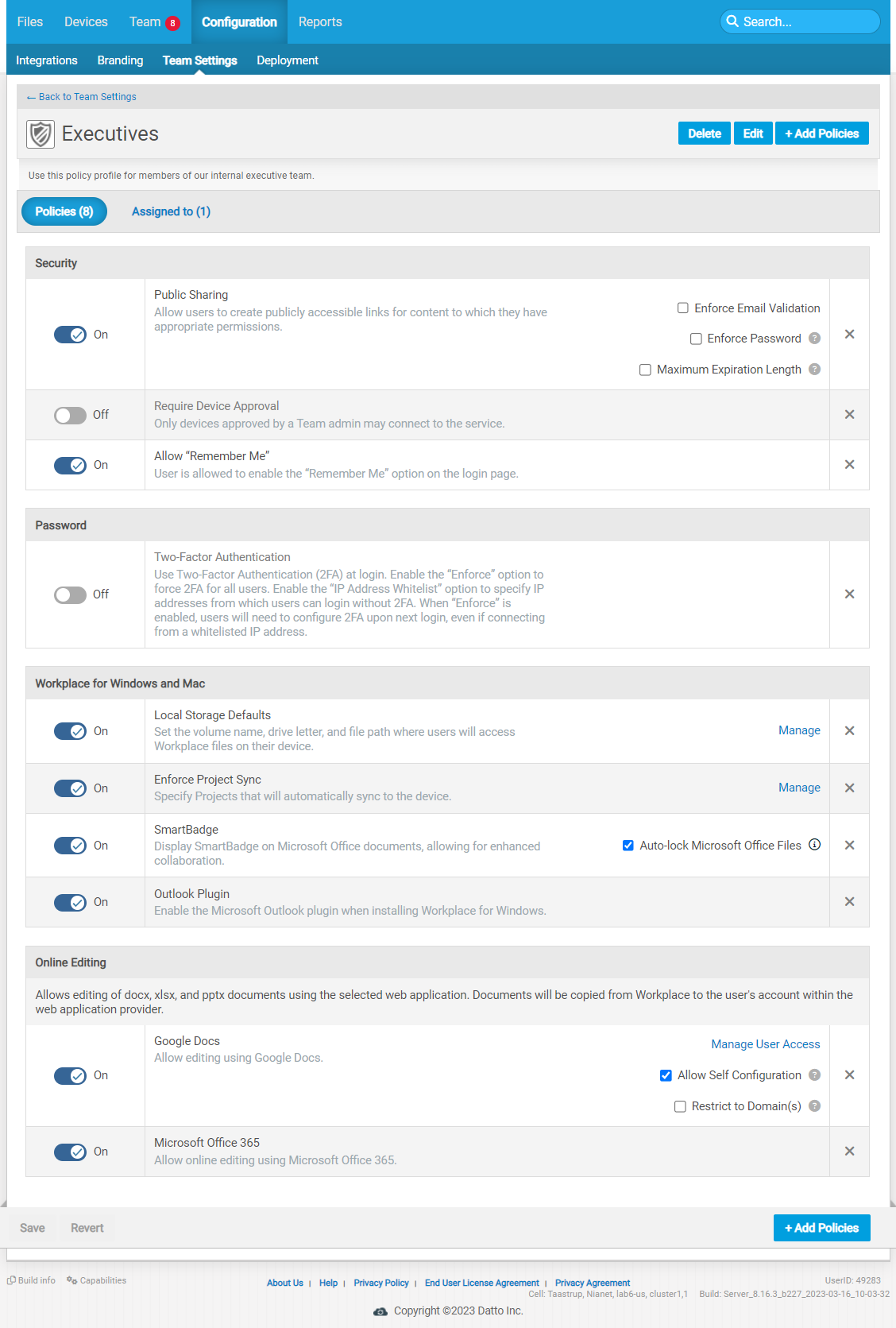In this on-screen image, the uppermost section features a prominent blue banner with various tabs, including "Files," "Devices," and a trash icon followed by a red circle. Adjacent to these is a configuration icon and a reports icon. Positioned in the upper right corner is a search bar. Below the blue banner, there are additional selectable tabs. Moving further down, there is a section labelled "Executives" accompanied by an executives icon. On the right-hand side of this section are three tabs: "Delete," "Edit," and another tab that is difficult to discern due to its small size, but possibly related to adding items. Beneath these tabs is a blue "Follow" icon. The central area of the screen displays various security measures. This section starts with a light gray banner bearing the word "Security" at its beginning. Under "Security," there are multiple tabs to choose from, enabling the user to toggle different security features on and off. Finally, a "Password" tab appears beneath the security options, allowing users to manage password settings.